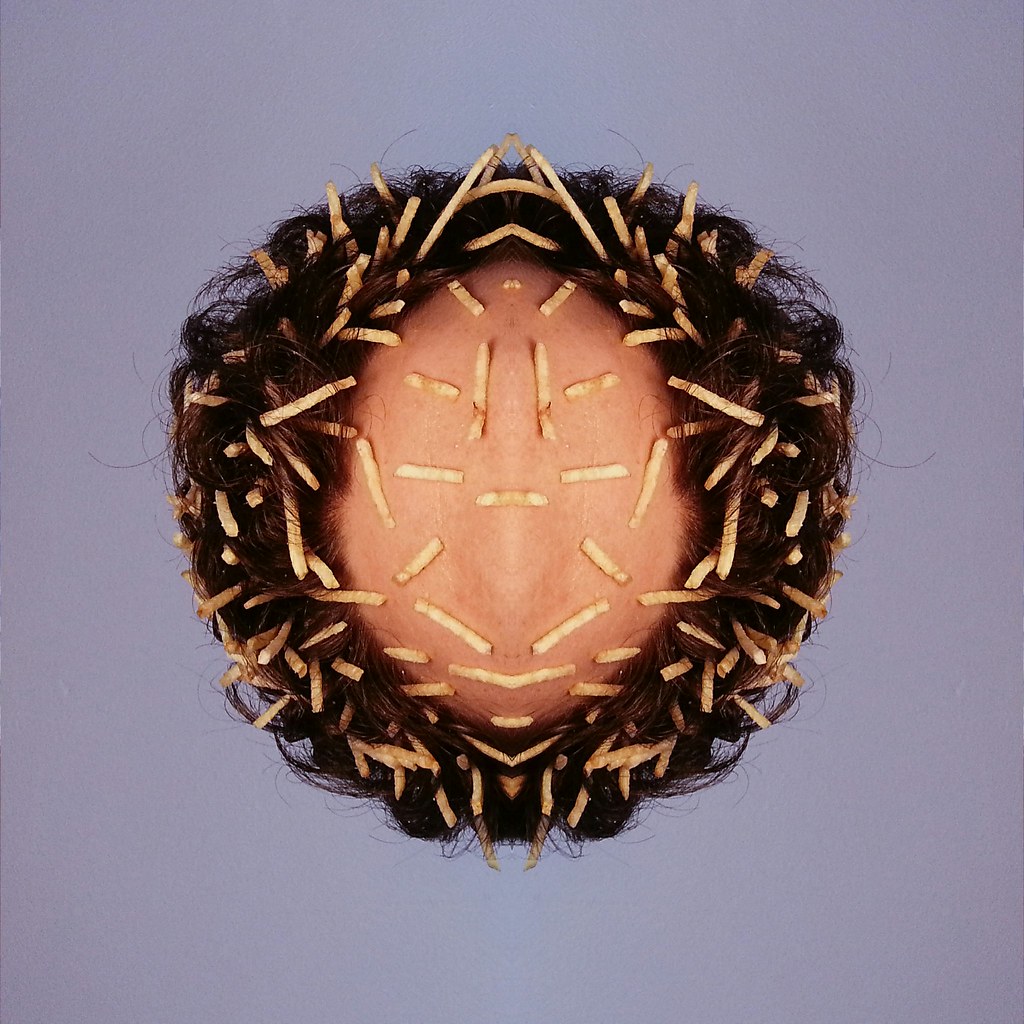The image presents a surreal, top-down view of the top of a person's head, featuring a large bald or completely shaved area in the center. This central bald spot is encircled by thick, dark, curly hair that almost resembles a bird's nest. Intricately woven throughout the hair and scattered on the bald area are long, thin, golden brown objects that appear to be french fries or potato chip crisps. These fries are arranged in a somewhat symmetrical, geometric pattern, with some forming teepee-like shapes while others are randomly intertwined with the hair. The entire composition has a flat lavender or gray background that enhances the surrealist and reflective quality of the scene, making it appear almost as if a mirror effect is in play. The overall impression is one of an intriguing, almost bizarre aesthetic that blends elements of human anatomy with unexpected, whimsical details.